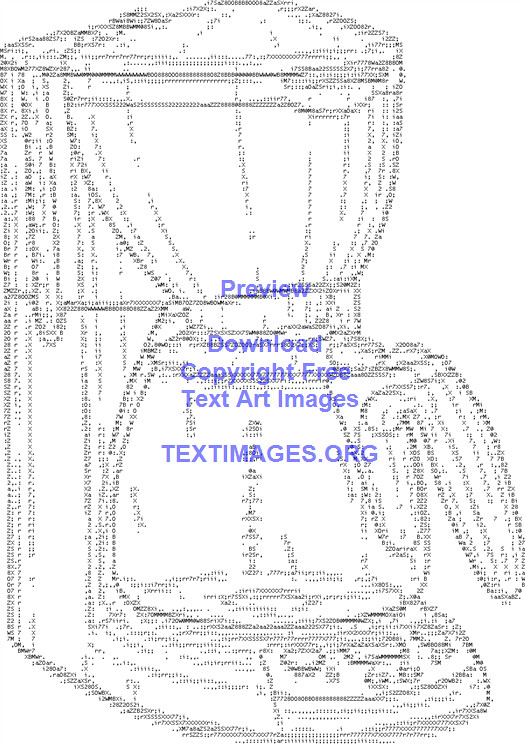This photo features a coffee maker, resembling the classic Mr. Coffee design, set against a white background. The coffee maker includes a visible coffee pot and filter compartment. Upon closer inspection, the entire image is composed of small letters and numbers, giving it a pixelated, text-art appearance. The coffee maker's contours look serrated and fuzzy due to the textural detailing. Overlaying the coffee maker image, in light blue font, are the words "preview," "download," "copyright free," "text art images," and "textimages.org," suggesting the image originates from a website specializing in text-based artwork.